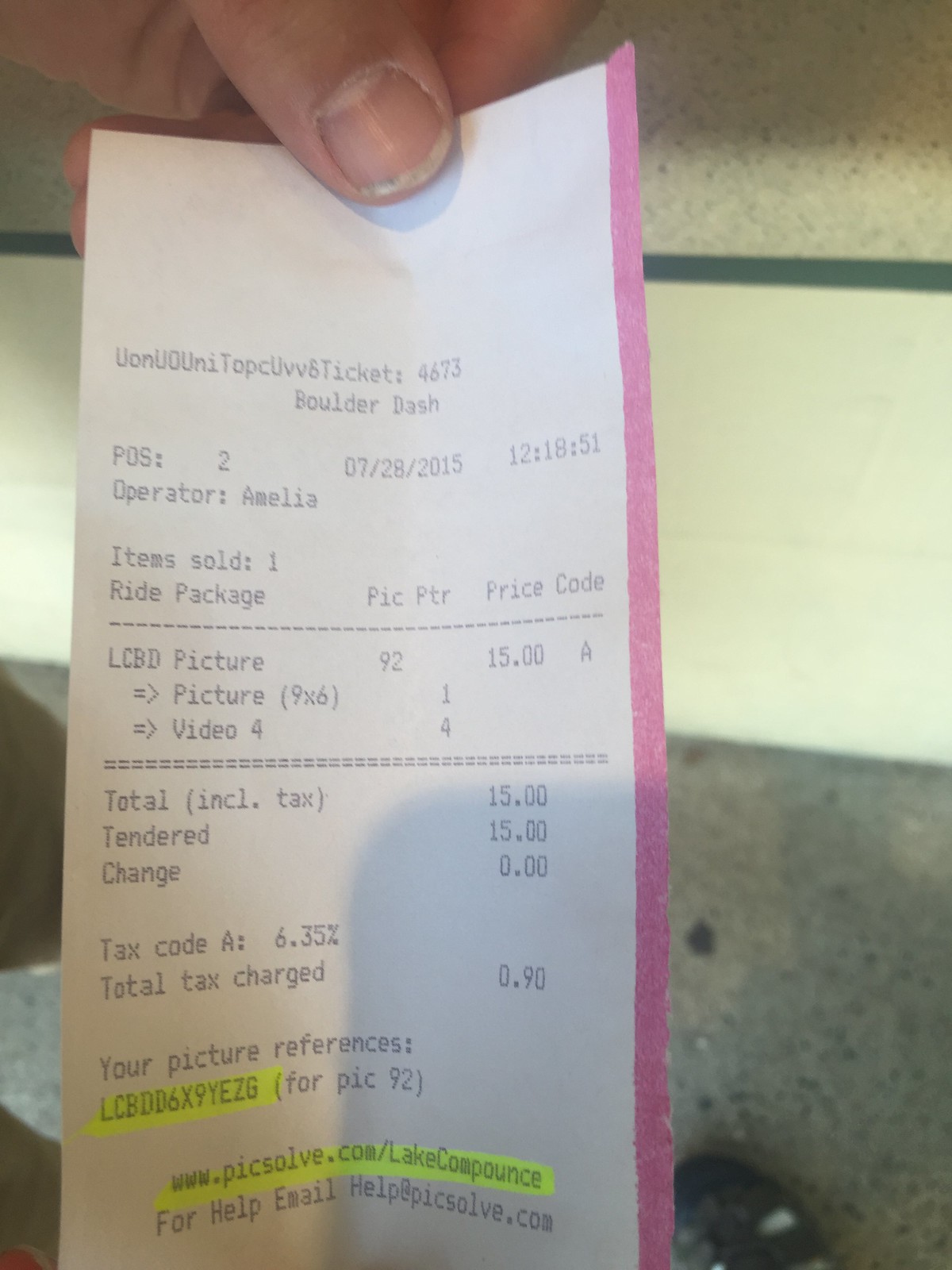This image shows a receipt with a tool roll that appears to be nearly depleted, indicated by a bright pink stripe along the right-hand side. The receipt lists an "Items Sold" section with a "Ride Package" priced at an unspecified currency. The total amount due is 15 units of this unnamed currency. Further down, the receipt mentions "Your Picture Preference" followed by a code in brackets: [PIC 92]. Below this, a URL is provided: www.picsolve.co/lakecompound.